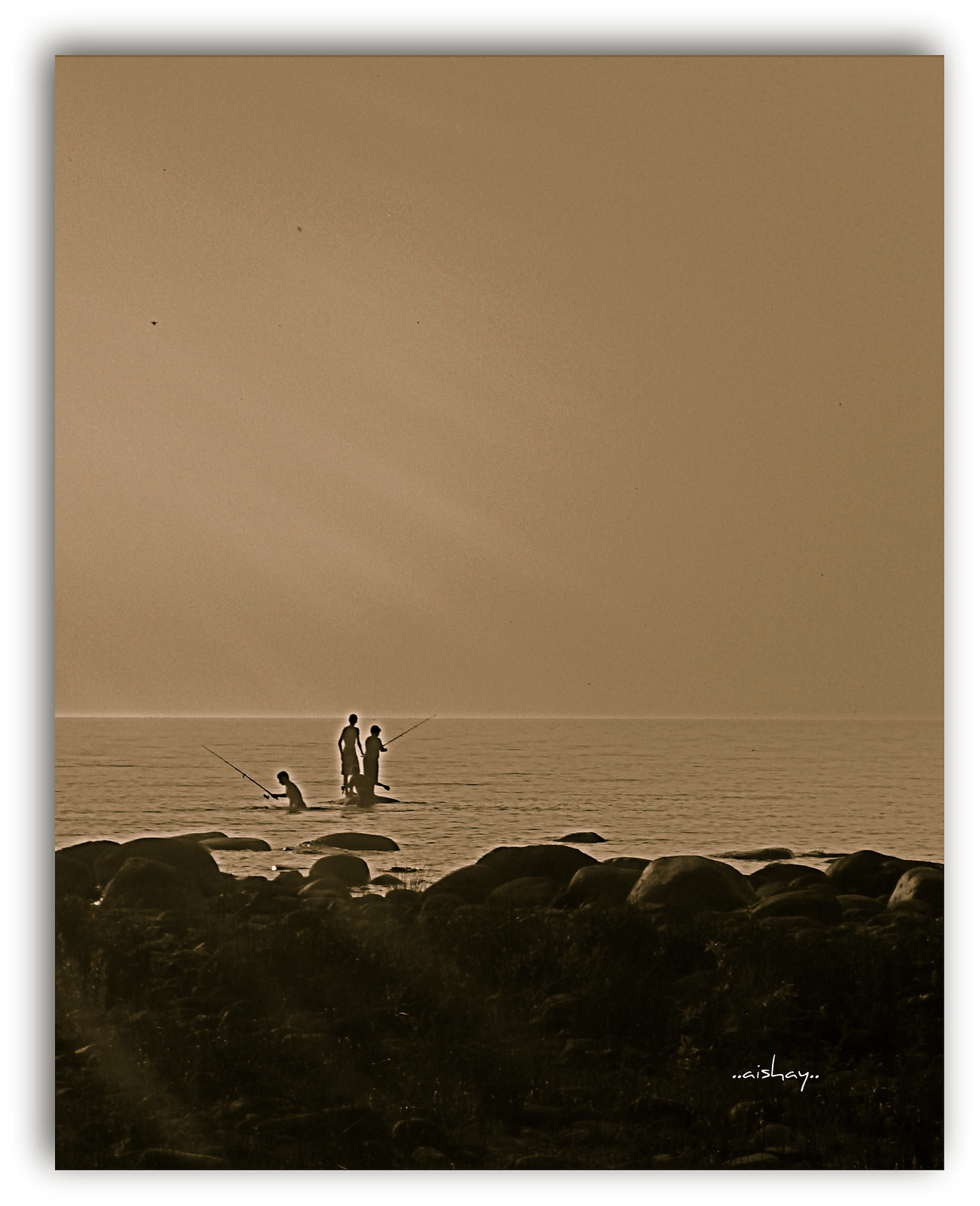The image depicts a serene scene, likely captured in a sepia-toned photograph or painting printed on canvas. In the foreground, a collection of rocks leads the viewer's eyes to a calm body of water, suggesting it is probably a lake due to the absence of wave action. The photo, illuminated by rays of sunlight streaming in from the upper left corner, portrays four boys engaged in fishing. Two boys are positioned on a large rock jutting out from the water, while another two appear partially submerged in the lake, actively participating in the fishing activity. The peaceful ambiance of the sunny day adds to the idyllic nature of the scene. At the bottom right corner of the image, there's a signature, possibly reading "AISHAYI," marked with two dots on either side and written in white letters, indicating the artist or photographer's name.